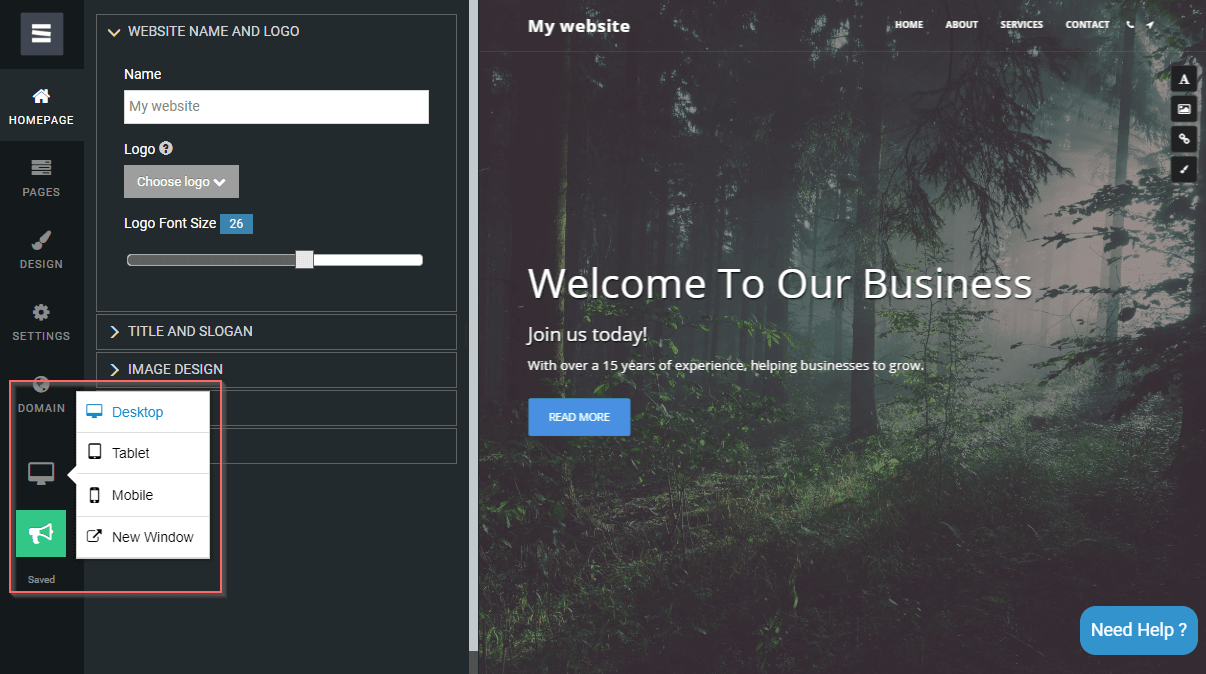A screenshot showcasing a website building interface, divided into two segments against a black background. The left segment, smaller than the right, features a series of controls in white text. At the top, it displays "Website Name and Logo," followed by fields to input the website name. A text entry box, preset with "My Website" in gray, allows for custom input. Below, a "Choose Logo" button facilitates logo selection, alongside an option to adjust logo font size with a blue box displaying "26" and an adjustable slider. Further down, expandable menu items labeled "Title and Slogan" and "Image Design" are indicated by right-facing arrows. The left sidebar offers additional navigation options: Homepage, Pages, Design, Settings, Domain, and Saved.

The right segment, which is the preview and development area, shows the website under construction. At the top, "My Website" is prominently displayed, with navigation links for Home, Our Services, and Contact. The main website preview features a welcoming headline: "Welcome to Our Business," followed by a subheading that invites users to join, citing "over 15 years of experience helping businesses grow." A prominent blue "Read More" button is situated beneath the text.